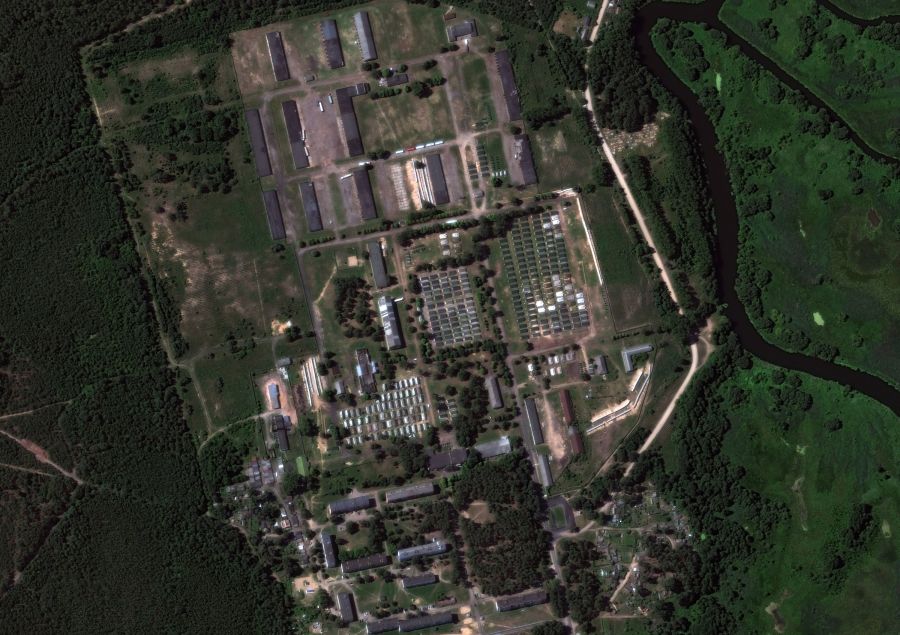This detailed satellite image captures the Belarus garrison from several thousand feet in the air. The garrison is characterized by its extensive greenery, with the winding lines of trees and patches of grass dominating the landscape. To the right, there's a river coursing through the area, while beige-colored dirt roads meander through the scene. The left side of the image shows a dense forest, its deep green hues indicating thick, bushy trees growing closely together.

In the center of the photo, rows of rectangular buildings and barracks are clearly visible, their roofs neatly aligned and suggesting a purposeful layout. Among these structures, some buildings appear to have divided roof lines, potentially indicating storage units or areas. Towards the upper center of the image, these elongated buildings resemble shipping containers in pattern and structure.

At the bottom of the image, an entrance area can be seen, with smaller buildings possibly designated as parking zones. These areas are also interspersed with clumps of trees, enhancing the overall tree-lined appearance of the garrison. Throughout the image, the repetitive, orderly placement of structures amid the lush surroundings presents a rural yet organized setup, devoid of conventional urban elements like paved roads or cars.